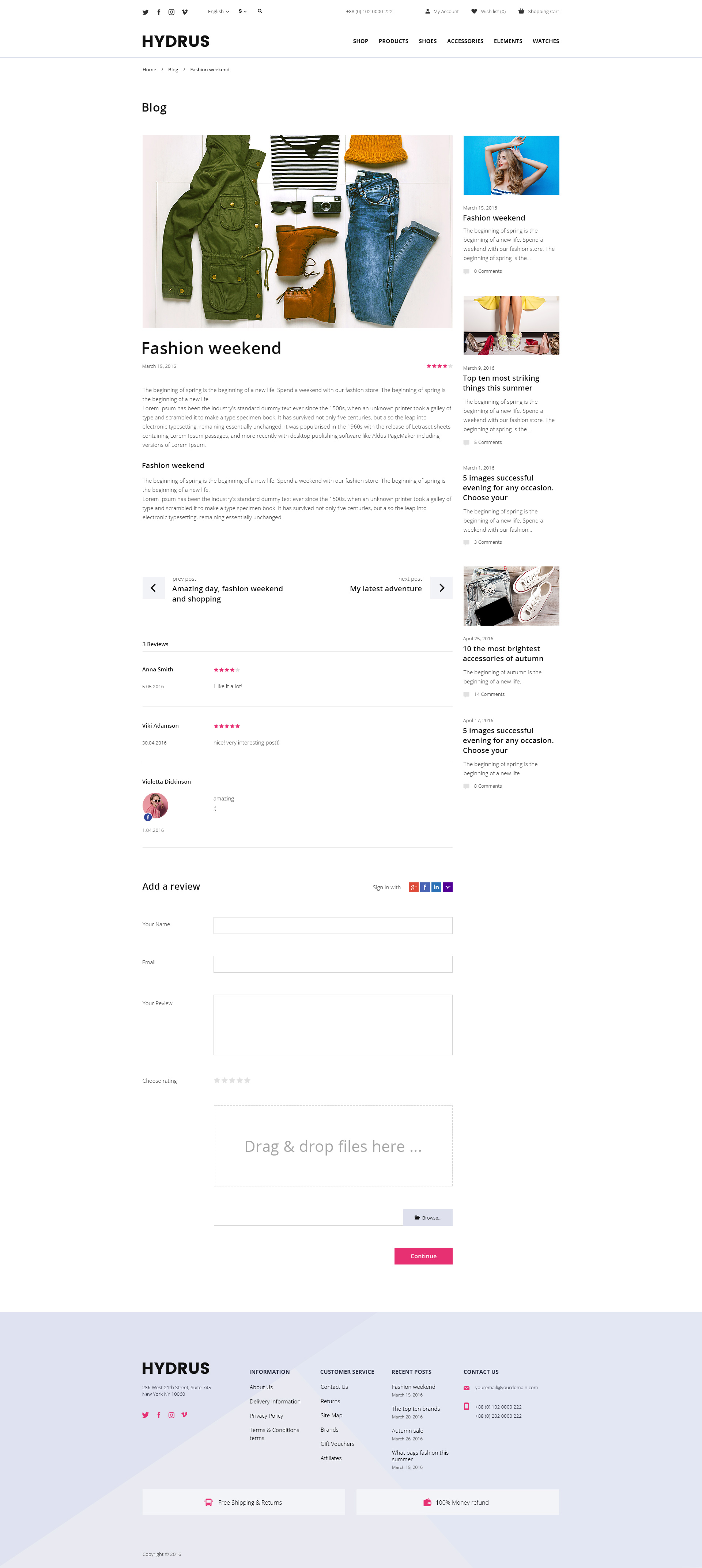The image appears to be a screen capture of a fashion website, possibly featuring a specific brand named "Hydrus." At the top, there are difficult-to-read fonts, with some text in bold black font spelling out "Hydrus." Above the brand name, there seem to be several social media icons in black.

Below the social media icons and brand name, there are multiple submenus, each represented by an icon. Moving down, there's another series of approximately six submenus followed by bold black text that is partially illegible, but clearly includes the words "Fashion Weekend."

An image below this text showcases an outfit ensemble including an olive green jacket, brown boots, blue denim jeans, black sunglasses, a black and white purse, and a mustard-colored clothing item. Underneath this, "Fashion Weekend" is followed by around two to three paragraphs of descriptive text.

Further down, there are more black text elements and additional submenus, some of which appear in pink, alongside others in black. There is a profile picture outlined in a pink circle, though this section is blurry.

On the right side of the image, there are several more photos. One features a woman with her hands up against a blue background, accompanied by a paragraph of text. Next to it, another image displays someone's legs, with two paragraphs of text beneath it. Additionally, there is an image of fabric with more accompanying text.

Towards the bottom, there are colorful social media icons in purple, blue, and orange. Several boxes appear near the bottom of the screen, including a pink and white box, and multiple gray boxes filled with text. The brand name "Hydrus" is repeated, surrounded by several submenus and clickable links, with some pink icons prominently displayed.

Overall, the screen capture is a detailed representation of a fashion-focused website, featuring brand elements, navigation menus, textual descriptions, and a variety of fashion-related images.